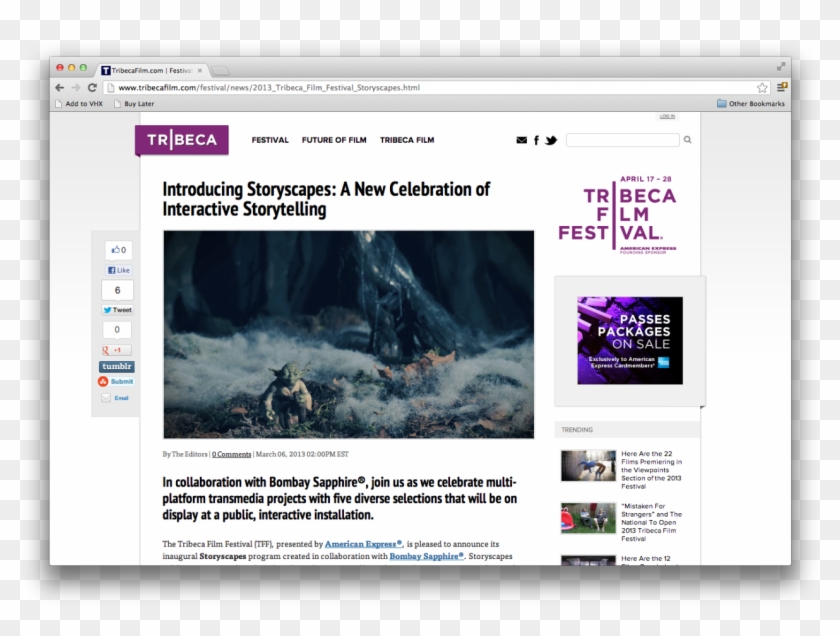The image depicts a MacBook screen displaying a webpage with a transparent background, as indicated by the grey and white checkerboard pattern. Toward the top left of the MacBook screen, the familiar macOS window control buttons—small red, yellow, and green circles—are visible, confirming that the device is indeed a MacBook. The webpage highlighted on the screen features a distinctive logo on the left side that reads "Tribeca," with an elongated "i" stylized to resemble clip art. The logo is set within a dark purple rectangle, and the text appears in white font.

To the right of the logo, the text "FESTIVAL, FUTURE OF FILM, TRIBECA FILM" is displayed in capitalized black letters, uniformly sized and aligned. Below this, a prominent, bold black headline announces: "Introducing Storyscapes: A New Celebration of Interactive Storytelling."

An image adjacent to the headline shows a figure that could be either Yoda or Baby Yoda, set against a backdrop that appears snowy or cloudy. To the right of this image, there is an advertisement bordered in a thick light grey frame. The ad's text states "Passes Packages on Sale," with the phrase "Tribeca Film Festival" prominently displayed above it in dark purple, fully capitalized font. The logo again features the elongated "i."

At the top right corner of the website, smaller capitalized purple text indicates the event dates as "APRIL 17th TO THE 28th."